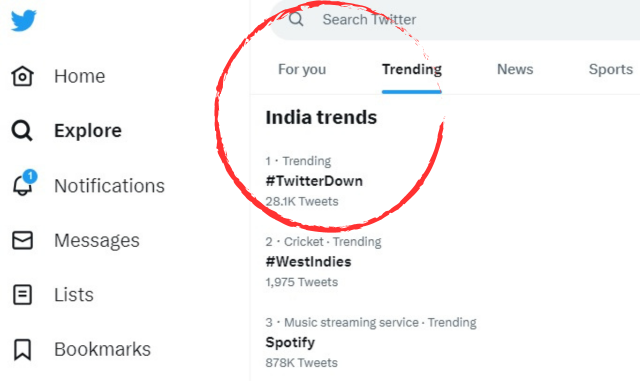The image depicts a user interface of a social media platform, likely Twitter. 

On the left side, there is a blue bird icon representing Twitter. Below this, various menu options are listed in black text. These options include "Home," "Explore," "Notifications," which is accompanied by an outline of a bell in black and white with a blue circle containing a number. Following "Notifications" are "Messages," "Lists," and "Bookmarks."

To the right of these menu options is a vertical gray line. Beyond this line, there is a horizontally truncated gray oval search box with a magnifying glass icon inside it. The text inside the search box reads "Search Twitter" in gray. Below the search box is the text "Forward" in gray, and next to it, "Trending" in black, underlined in blue. Continuing in gray are the words "News" and "Sports."

Further down, a horizontal gray line runs across the interface. Below this line, the text "India Trends" is displayed in black. The trending topics are listed beneath. The first trend is labeled as "number one Trending" in gray, followed by "#TwitterDown" in black with "28.1k Tweets" in gray. 

A red circle seems to encompass the area from the trending list up to the search bar, enclosing the terms "For You" and "Trending."

The second trending topic under "Cricket-Trending" reads "#WatchIndies" in black, with "1,975 Tweets" noted in gray. 

The third trend listed is "Music Streaming" and "Service Trending," with "Spotify" mentioned in black accompanied by "878k Tweets" in gray.